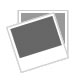The image showcases a detailed gray and white toy dinosaur set on a marble surface with intricate black veining. The dinosaur, predominantly gray with a white underbelly and neck, stands front and center in the horizontal photograph. Its long, wrinkled neck, resembling that of an elephant, twists backward, partially obscuring its face but revealing its eye and the side of its mouth. The dinosaur's legs, also similar to an elephant's, end in black-tipped toes. Draped over its back is a brown leather saddle with white trim, suggestive of it being rideable. The background includes a shiny, white wall, adding to the overall monochromatic aesthetic of the scene.